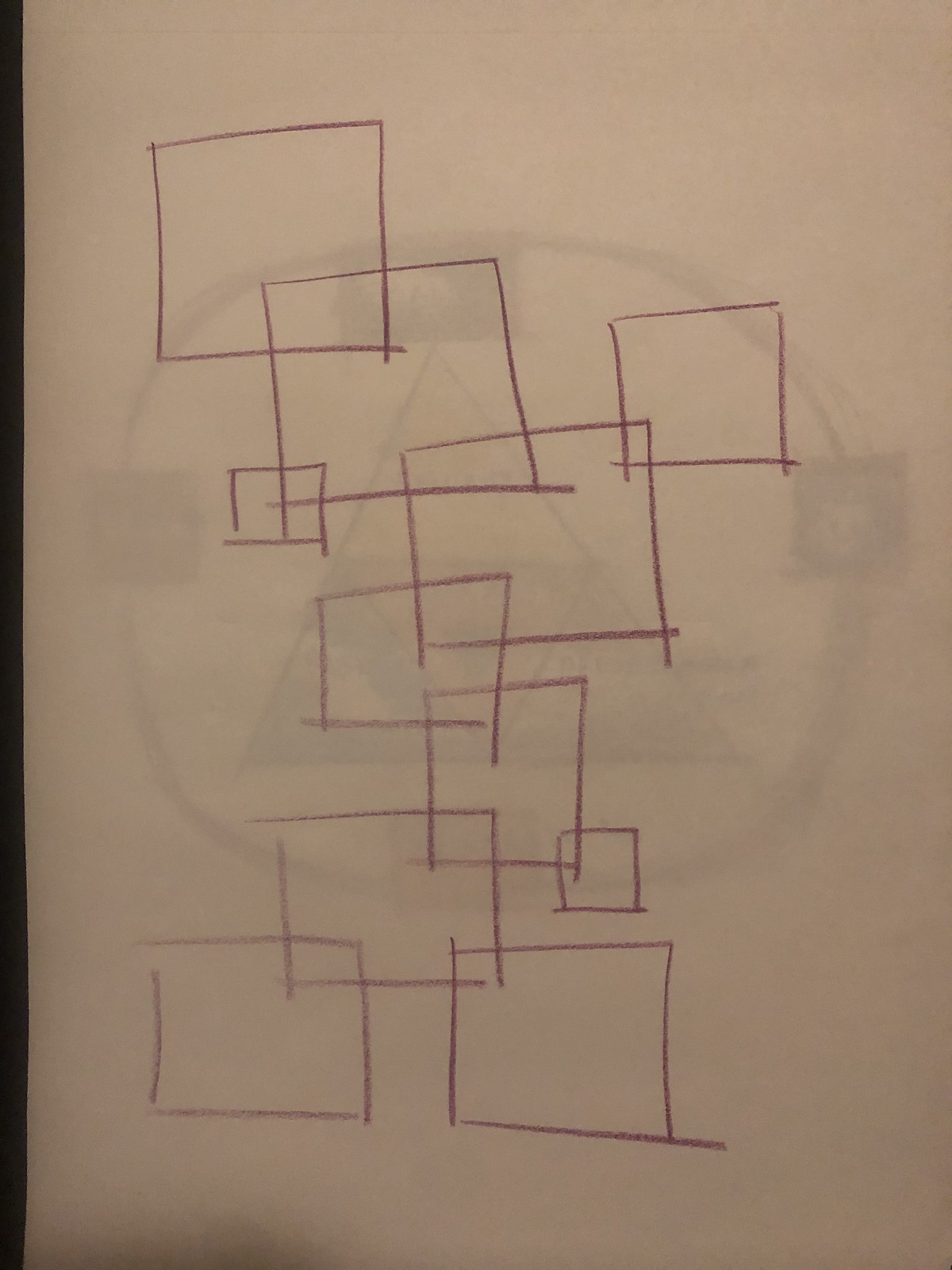The drawing on a large sheet of paper features an array of hastily sketched squares of various sizes, many of which overlap. In the upper left corner, a square begins the series, with another square overlapping on the bottom corner. A smaller square overlaps the bottom left corner of the initial square, while a larger one overlaps the bottom right corner. A medium-sized square intersects the upper right corner of this larger square. Another square overlaps the bottom left corner, also encroaching upon the upper left corner of the square below. To the side, a small square overlaps the bottom right corner, and a larger one overlaps the bottom left corner. Two more squares emerge from this section, one overlapping the bottom right corner and the other, the bottom left corner. 

In the background, faintly visible through the paper, there is an intriguing outline on the subsequent page. This outline resembles a large circle encompassing a Triforce symbol, with three to four smaller boxes positioned around it, each containing indistinguishable images. The entire scene seems to be rendered in shades of green, adding an additional layer of complexity, though this coloration might be an effect of viewing through the translucent paper.